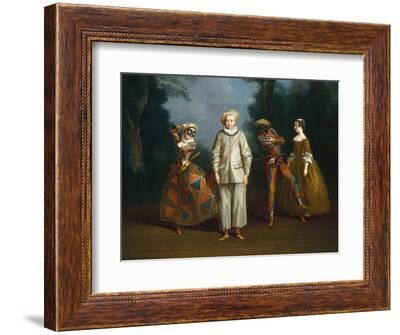This is a detailed image of a framed artwork, likely a print of a famous painting, with a simple brown wooden frame and white matting. The painting showcases four figures standing outdoors, set against a dark forest background with a gray-blue sky. The central figure, dressed in a white jacket and white pants, is ambiguous in gender. To the left, a woman in a red, patterned dress and a black mask appears somewhat flirtatious, almost performing a dance-like gesture with one hand raised to her head. On the right, another woman, wearing a green dress and a headpiece, engages in conversation with a man dressed in a reddish-beige outfit that resembles a jumpsuit, who leans back slightly as he listens. The overall scene exudes an eerie, Renaissance-inspired vibe, with elements that hint towards a masked ball or some form of dramatic interaction.